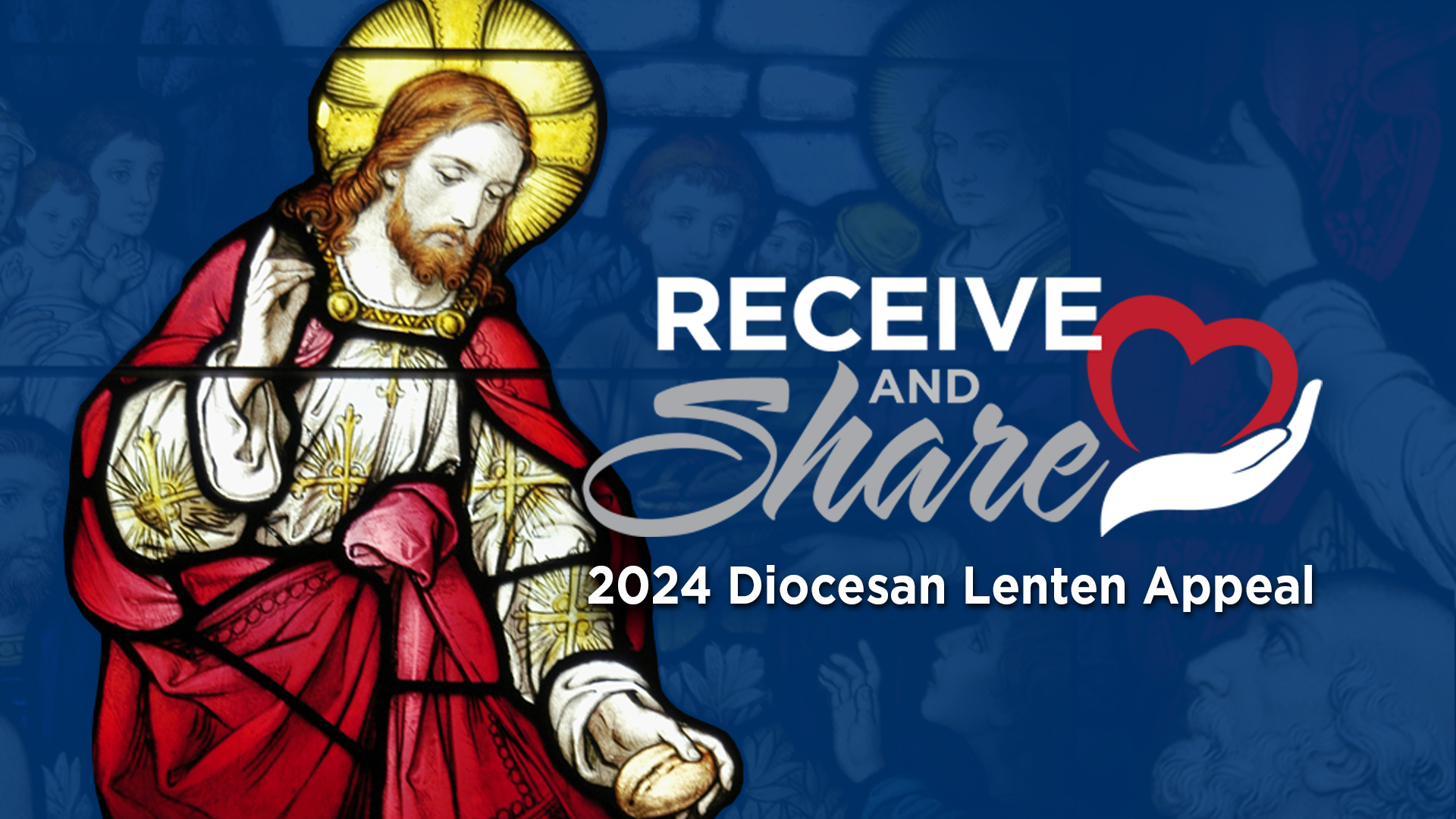The image depicts an intricately designed illustration reminiscent of a stained glass window, featuring Jesus Christ prominently on the left. Jesus has a yellow halo around his head, and his attire includes a red cape, a white and gold robe adorned with crosses, and a draping white garment. He is shown holding bread in his left hand. The background is a blue hue with watermark images giving a subtle texture. To the right side of Jesus, the words “Receive” in bold white letters and “Share” in italicized gray letters are prominently displayed. Below this text is the logo of an outstretched hand cradling a red heart. At the very bottom, the inscription reads “2024 Diocesan Lenten Appeal,” highlighting the religious context and timeframe of the image.